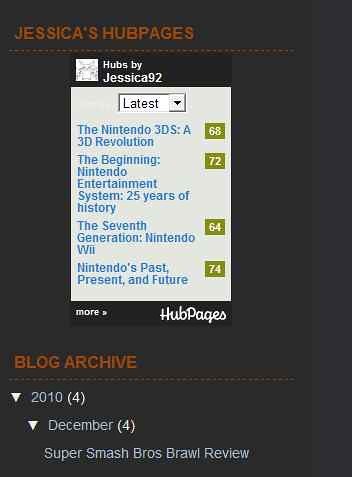The image depicts a screenshot of a webpage titled "Jessica's Hub Pages" in bold orange capital letters at the top, underlined by a dashed line. Within the page, there's a smaller rectangle labeled "Hubs by Jessica92" with a drop-down menu set to "Latest," showcasing Jessica's most recent articles. The highlighted hubs include reviews and retrospectives such as "Nintendo 3DS: A 3D Revolution," "The Beginning of Nintendo Entertainment System: 25 Years of History," "The 7th Generation: Nintendo Wii," and "Nintendo's Past, Present, and Future." Below this section, there is another labeled "Blog Archive" in orange, featuring a drop-down box for the year 2010 expanded to show four entries, the first being a "Super Smash Brothers Brawl Review." The background of the image is dark gray, while the titles and text are in contrasting colors, with some links in blue and important headings in orange.